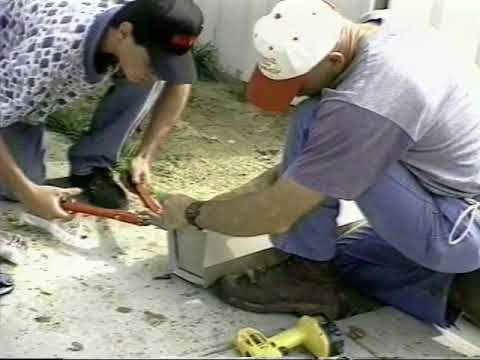The image captures a moment of hands-on work with a nostalgic feel, likely from the late 80s to early 2000s. The square-shaped photo, taken outdoors under natural light, features two men engrossed in their task, kneeling on the dirt-covered ground. On the right, a younger man with lighter skin wears blue jeans, brown boots, a gray short-sleeved t-shirt, and a white ball cap with a red brim. He's firmly holding a metal beam or gutter. Beside him lies a yellow power tool, possibly a hand drill. On the left, an older man, potentially his co-worker or father, sports a black hat with red lettering, a white and blue shirt, blue jeans, and black boots. He holds a large red wrench, cutting into the beam or gutter. The image, while slightly obstructed by the men's arms, vividly displays their collaborative effort amidst the timeless backdrop of manual labor.